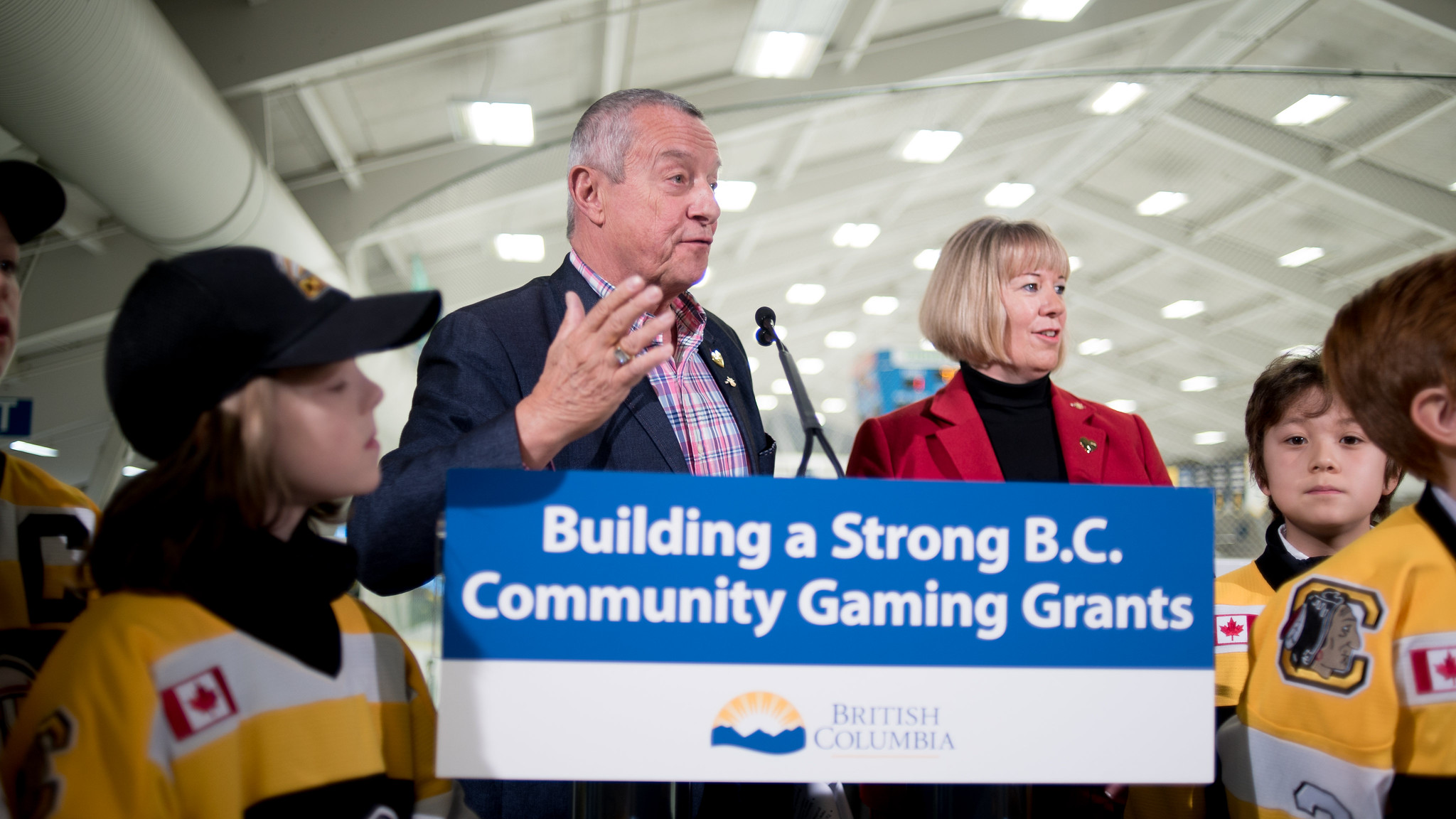The image depicts the inside of a hockey rink with metal rafters and fluorescent lighting. Central to the scene is a podium adorned with a banner that reads "Building a Strong BC Community Gaming Grants" in white text on a blue background, accompanied by a logo for British Columbia in blue and yellow on a white section of the banner. A man in a blue sport coat and a blue and red checked shirt is speaking into the microphone; he has short hair and gestures with one hand. Next to him on his right stands a blonde woman with short, chanel-style hair, wearing a black turtleneck and a red blazer. Surrounding them, especially in the bottom corners of the image, are several children dressed in yellow, white, and black hockey jerseys emblazoned with the Canadian flag. The scene suggests an award presentation or community event supported by the British Columbian gaming grants program.